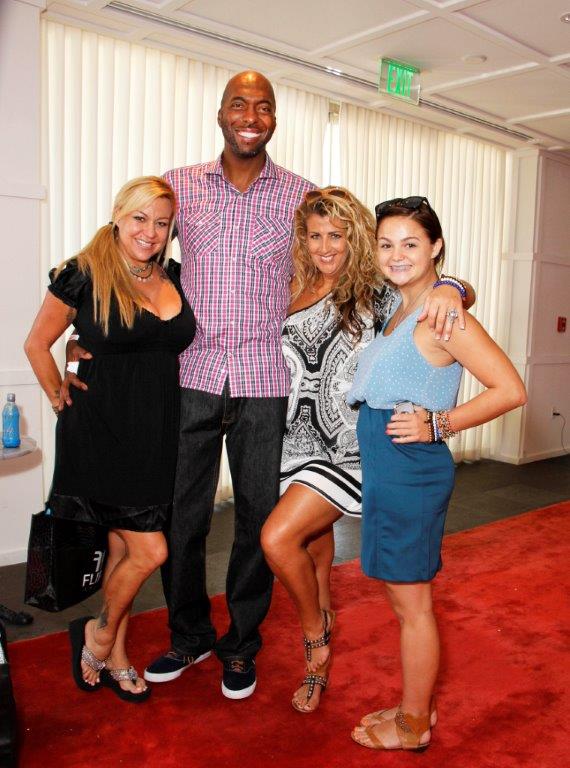In this photograph, four people are standing inside a room adorned with a red carpet. The group is composed of one man and three women, positioned as follows: 

On the far left is a woman dressed in a knee-length black dress paired with jeweled sandals. She has long blonde hair cascading down to her chest and is bending her right knee so it touches the man next to her. She has her hand behind her waist. Next to her, on her right, stands a very tall man wearing a checkered reddish-purplish button-down collar shirt, blue jeans, and black sneakers. He has his arm around the woman in the black dress and his other arm around the two other women to his right.

To the right of the man is a woman donned in a black and white mini dress. She is posing with her left knee lifted in the air and wearing sandals. Lastly, on the far right, is a woman in a light blue tank top and a blue skirt, with her arm placed on her waist. All four individuals are smiling and looking towards the camera.

The backdrop features a large window draped with white curtains and vertical shades, set against pristine white walls and a white ceiling. An exit sign is visible, indicating that the room is likely located within a public building.